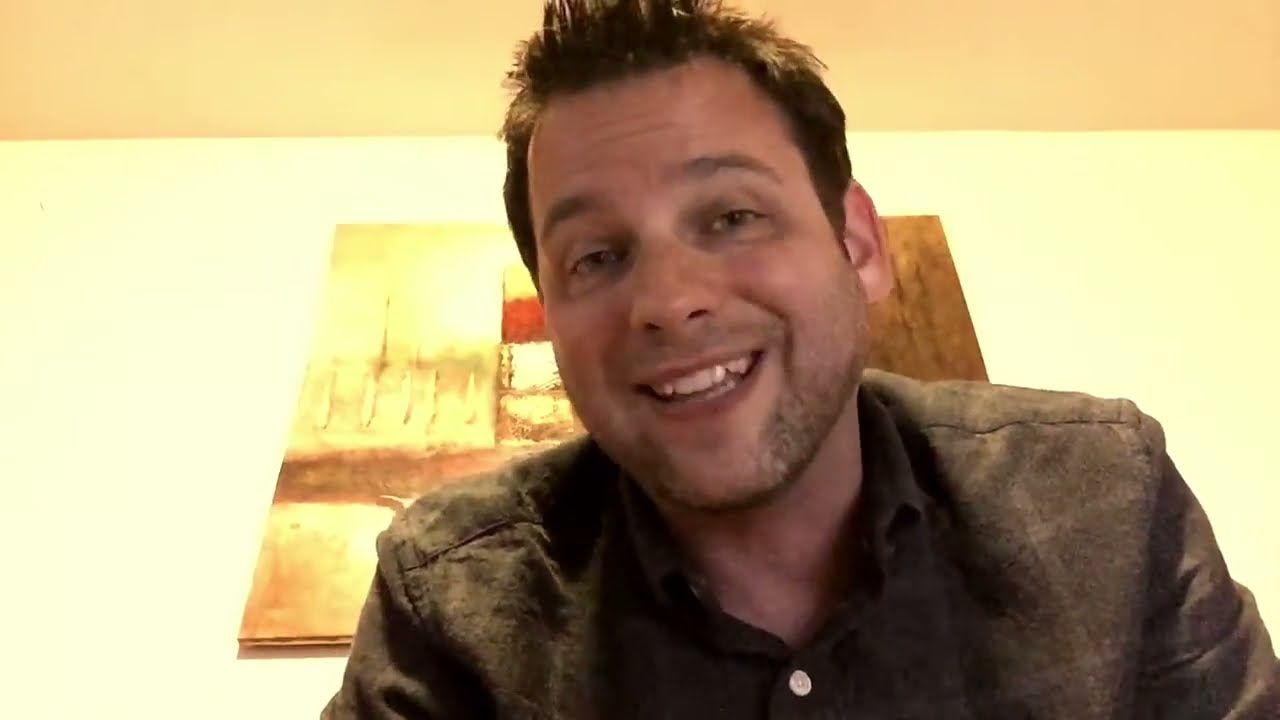The image captures a smiling Caucasian man with short to medium brown, spiky hair that is neatly trimmed around his ears. He has a fuzzy, short beard, resembling a five o'clock shadow. His head is tilted slightly to the left, and his open-mouth smile reveals his teeth. He appears to be engaging with a camera, possibly on a video call, suggesting a relaxed, conversational setting. The man is dressed in a brown button-down jacket, fastened with a single button at the base of his neck. Behind him, the background features a yellow wall that transitions to orange towards the top. A rectangular picture frame with various square images, including a mix of yellow, red, and brown colors, as well as a distinct brown section in the upper right corner, adorns the wall. The overall ambiance is warm, with a modern yet rustic aesthetic.